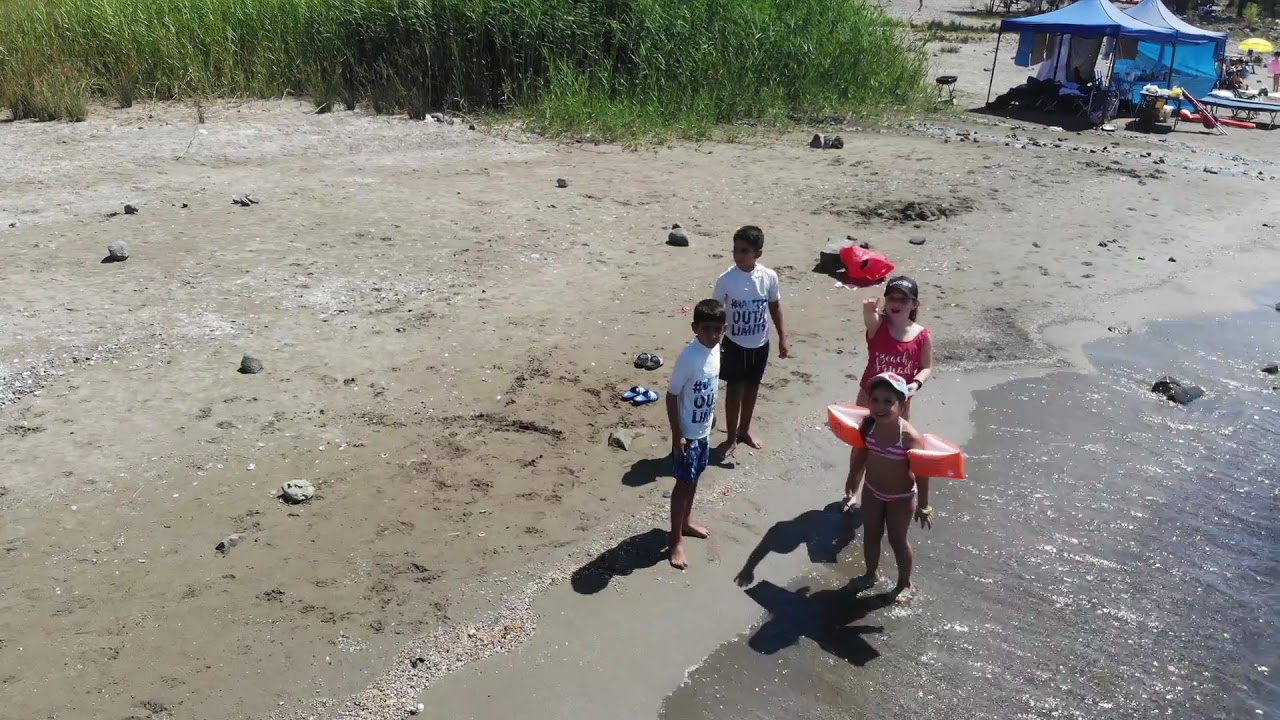In this detailed aerial photograph taken during the daytime, four children are playing at the edge of a beach. The beach, characterized by its clay and grayish soil, merges seamlessly into a flat, sandy expanse strewn with rocks and the occasional footprint. Just where the water meets the land, the children—two girls and two boys, presumably around seven or eight years old—are joyfully engaged.

The two boys stand to the left, each clad in white short-sleeved shirts adorned with blue prints, complemented by blue swim trunks. They both have dark, short hair. To the right, the two girls, both wearing baseball caps, are closer to the water. One girl with a striped bikini and arm floaties stands with her feet submerged, while the other, wearing a red tank top and a hat, straddles the shoreline with one foot in the water and the other on the sand.

In the background, lush green grass, about three to four feet tall, frames the scene, separating the beach from the more distant activities. Blue canopy tents are pitched in the upper right corner of the image, with people congregating underneath and around them. Further still, a yellow umbrella marks another gathering spot, enhancing the lively atmosphere of the beach. The sun shines brightly, casting reflections off the water and illuminating this vibrant tableau of a beach day filled with laughter and play.